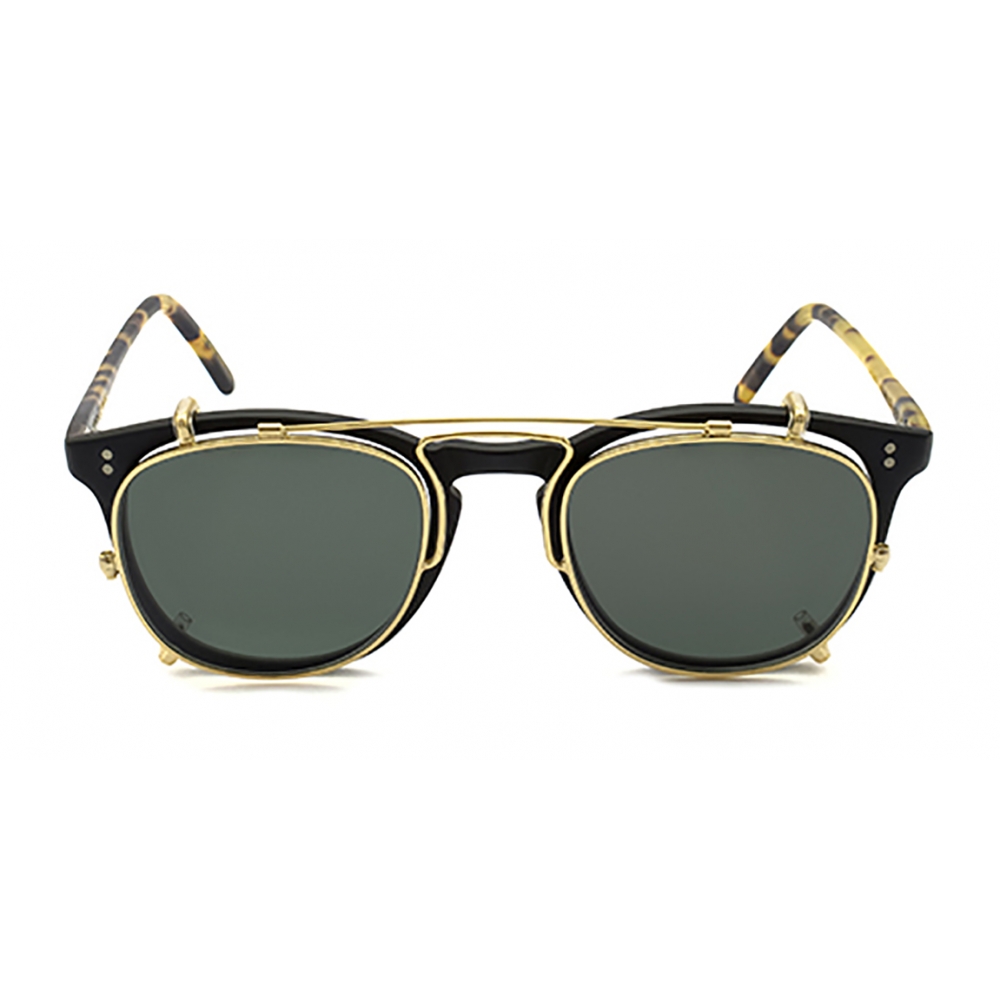The image is a highly detailed photograph of a distinctive pair of sunglasses resting on a white surface against a white background. The sunglasses feature a classical black frame with a dark, thick rim and very dark gray lenses. The arms of the glasses exhibit a tortoise shell pattern in black and tan, creating a striking contrast. Adding a unique element, the sunglasses incorporate a removable aviator-style golden metallic insert that attaches to the frame with visible screws. This insert consists of golden hooks that wrap around the top edges of the black frame, merging the classical and aviator styles into a cohesive, elegant design. The shadow of the sunglasses adds a touch of depth, enhancing the visual composition of the image.